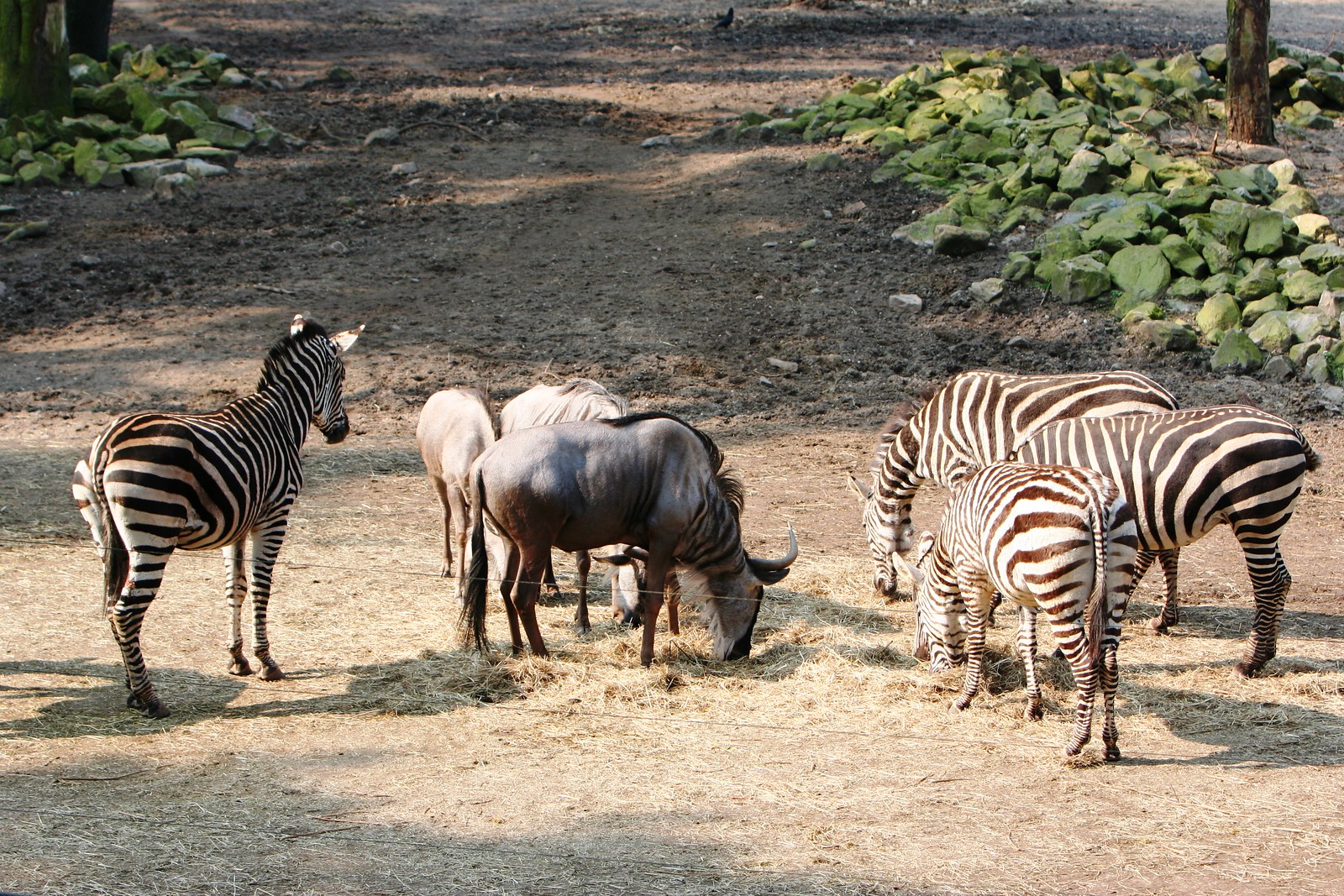The image depicts a grassy field with brown grass, inhabited by a variety of animals. On the right side, there are three zebras grazing, while another zebra stands off to the far left. In the middle background, there are three horses, one of which intriguingly has stripes around its neck, giving it a zebra-like appearance. In the foreground, there is a horned animal, possibly a bull. The field transitions into a rocky area with large, greenish rocks on both the left and right sides, likely covered in moss. Sparse trees are visible, with one tree trunk on the far left and another on the far right. The sun is shining brightly, casting significant shadows across the scene, especially over parts of the dirt pathway in the rocky area behind the animals.